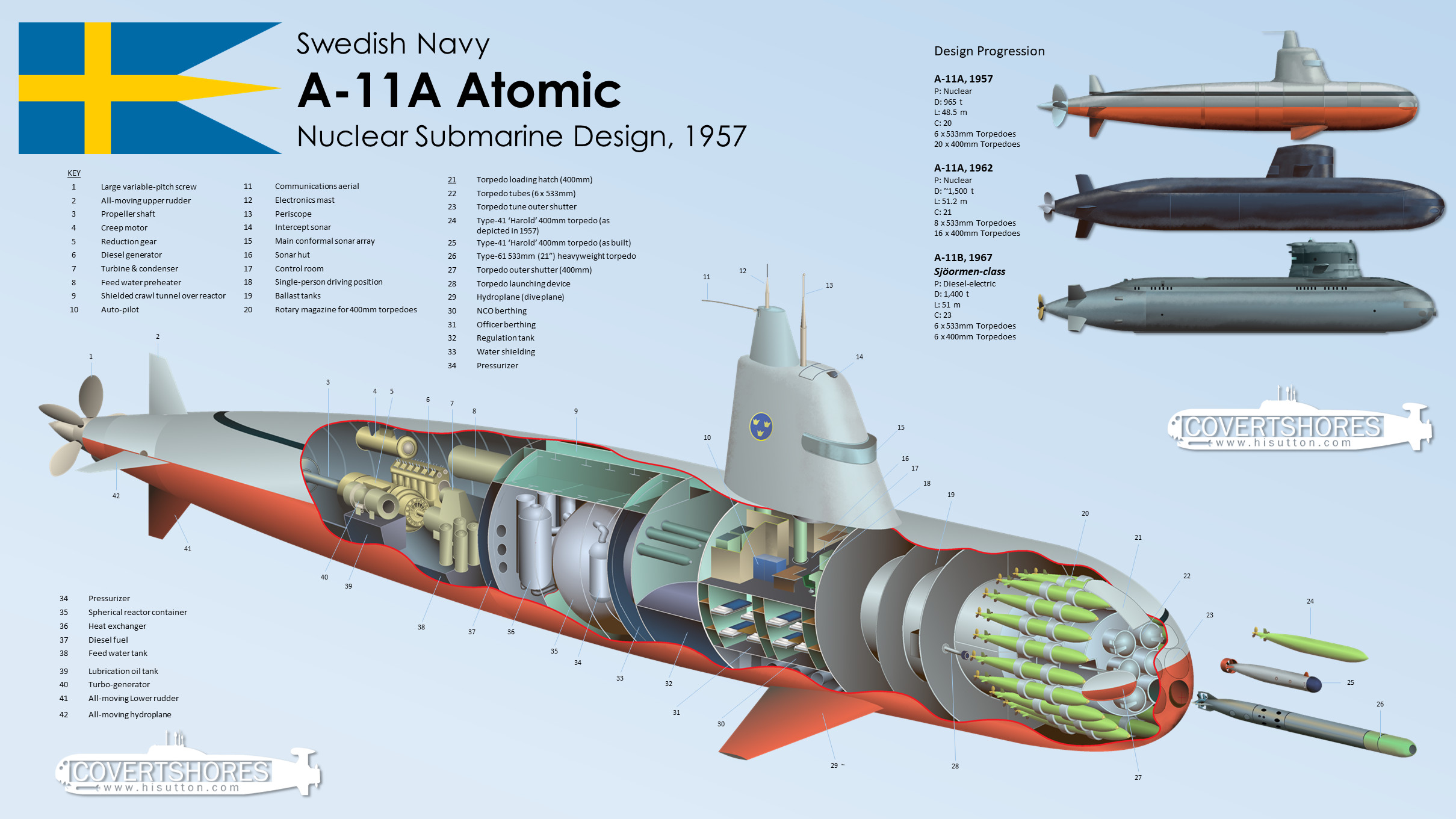The image is a detailed schematic poster of the Swedish Navy's A-11A Atomic Nuclear Submarine, designed in 1957. The top left corner features a Swedish flag with blue and yellow colors, alongside the title "Swedish Navy A-11A Atomic Nuclear Submarine Design, 1957." Below the title is a main design illustrating the submarine, with both the exterior and interior visible. The exterior of the submarine is white with orange trim. The interior view reveals an intricate design focused on the engine and various components, each meticulously numbered. There’s also a glossary and fine-print text outlining the components, although it is too small to read. Additionally, the top right corner showcases three different submarine iterations in orange, blue, and gray, illustrating design progressions. This poster resembles a museum exhibit sign, providing an educational and historical overview of the submarine’s design.